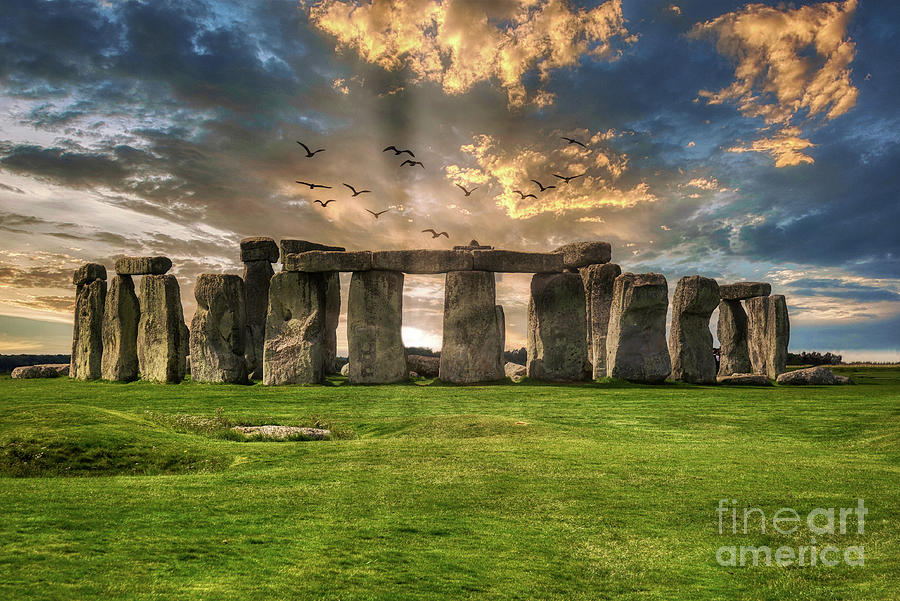This professionally taken photograph of Stonehenge captures the stunning ancient stone monument in a wide shot. Stonehenge is centered, with its iconic large vertical stones forming a circle, some topped with horizontal stone blocks. The photograph showcases a well-maintained, open green field stretching before it, likely mowed short. Above Stonehenge, the sky is a picturesque mix of vibrant blues and golds, dotted with both white and dark clouds, creating a dynamic backdrop that almost seems alive. Birds are captured in flight, their silhouettes adding a sense of motion and life to the still image. The photo's bottom right corner bears a transparent watermark reading "Fine Art America." The overall color palette is rich and varied, featuring blues, greens, grays, blacks, and hints of oranges, making this image a visually arresting portrayal of one of history's most enigmatic sites.